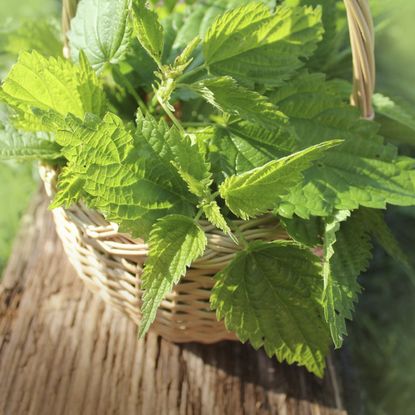In this close-up daytime photograph, a large green plant sits inside a light tan wicker basket, which features a visible handle extending slightly to the right and top left. The basket rests on a light brown wooden beam, resembling a tree log, which stretches across the image. The plant, which occupies the central and upper part of the frame, showcases an array of vibrant green leaves without any flowers. The leaves vary in shades of green and some extend beyond the edges of the basket, reflecting light and creating a mixture of lighter and darker green hues. The surroundings include bright green grass and bushes that create a blurred, nature-like backdrop, contributing to the overall focus on the plant and its leaves. The image is captured from a slightly elevated perspective, looking down toward the plant, enhancing the clarity and detail of the plant and the wicker basket.